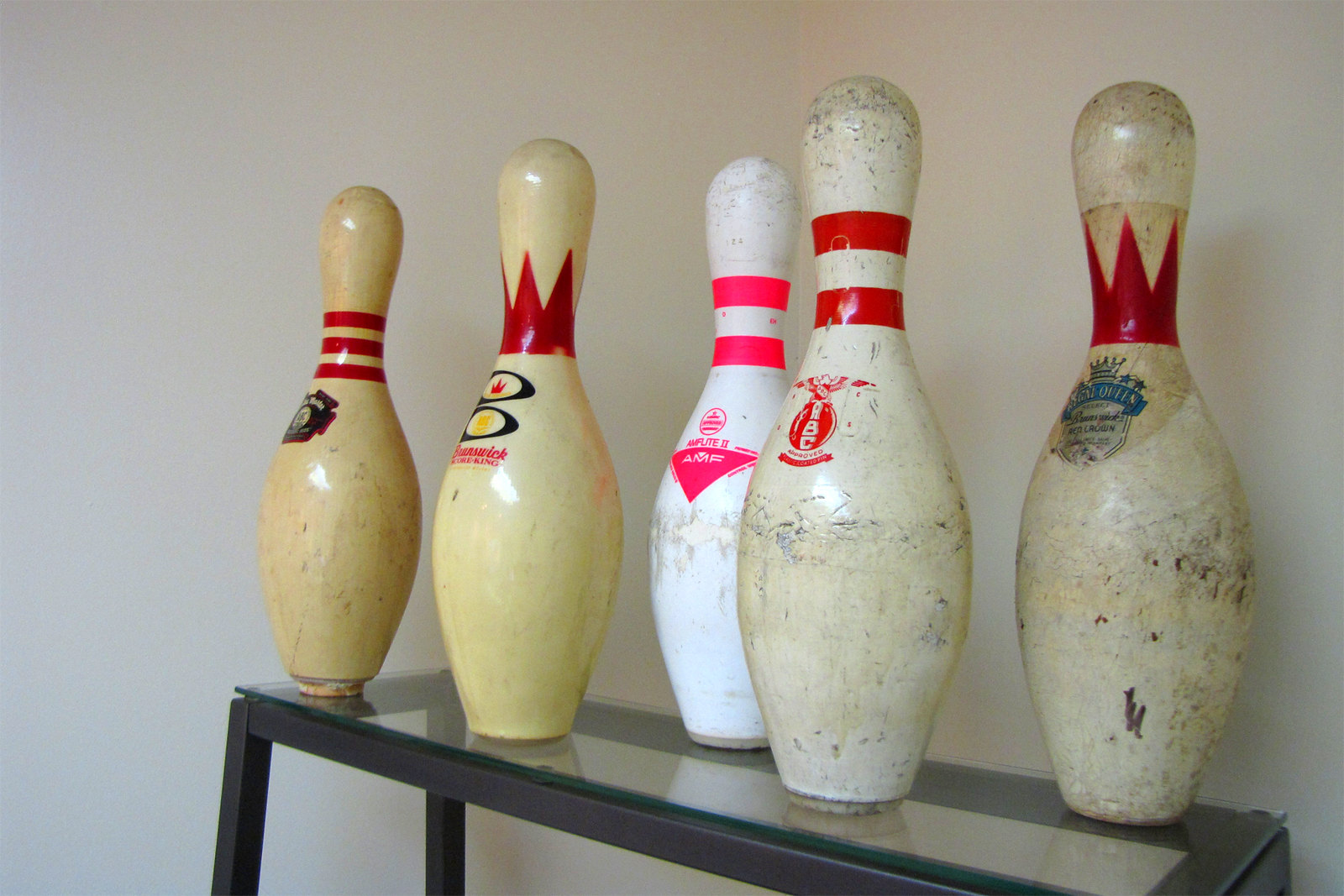This photograph showcases a minimalist glass-top shelf with a black metal frame set against a white wall. The shelf holds five distinct and aged bowling pins, each marked with unique designs and varying hues of white, accentuated by their wear and discoloration over time.

From left to right:
1. The first bowling pin stands out with its significantly yellowed and distressed appearance, featuring three horizontal red stripes at the narrowest part and a crest-like symbol on the front.
2. Next, a slightly less yellowed pin displays two blue oval logos with accompanying red text, crowned by a red-spiked emblem at its neck.
3. At the center, the whitest pin of the collection, albeit covered in black and brown marks, features vivid Dayglo decorations, including two red bands around the middle and a triangular logo near its widest part.
4. The fourth pin, though similarly whitish, is also marred by marks and discoloration, adorned with two red stripes and an obscure central logo.
5. The final pin, bearing a resemblance to the second, is primarily off-white and heavily distressed, topped with a red crown design at its neck and an ornate blue crown logo beneath.

Despite their varied conditions and decorations, all five pins share the commonality of age and history, contributing to a visually intriguing and story-rich display.